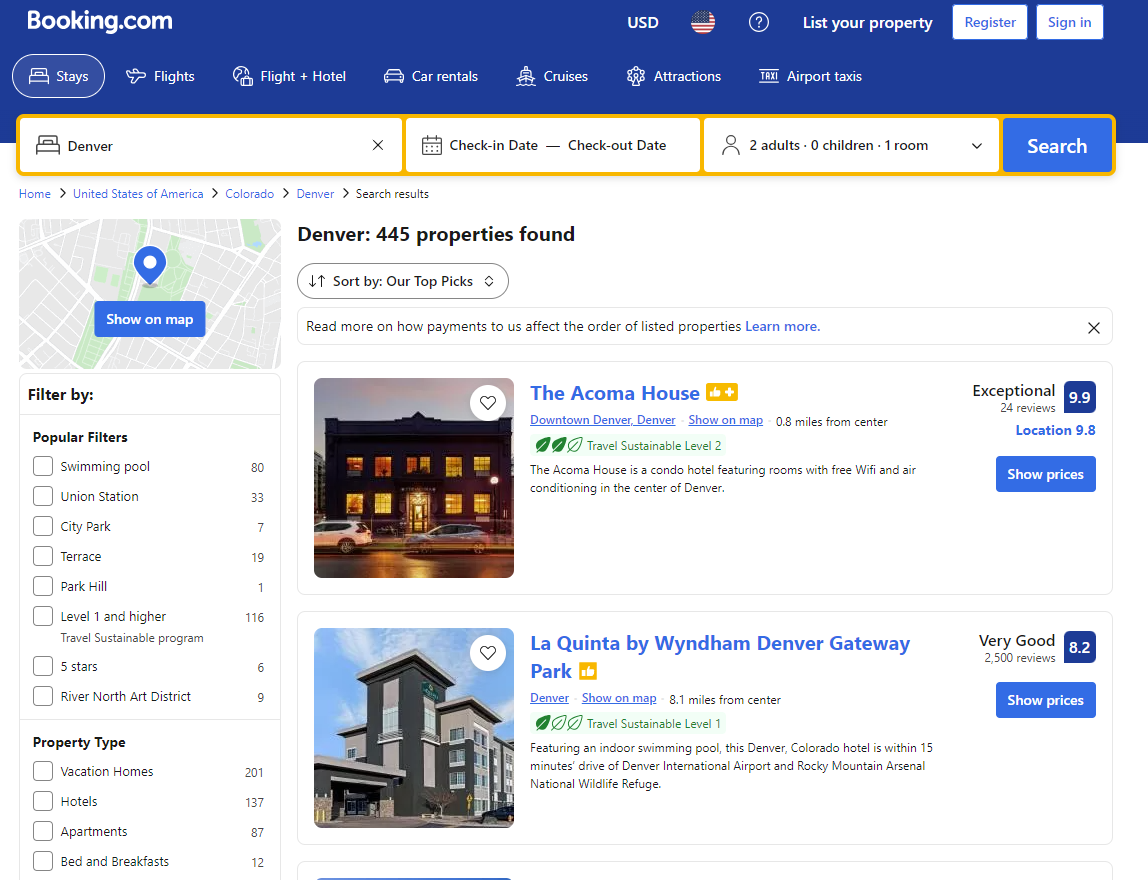**Caption:** A vibrant night scene featuring a bustling cityscape, where a prominent large building illuminated with yellow lights stands as the centerpiece. The foreground showcases parked cars, adding to the city's lively atmosphere. Beneath this main image is a secondary view highlighting a substantial gray building complemented by a sleek black tower on its side. This image conveys Denver's dynamic urban environment, with accommodations like LaQuinta by Wyndham, Denver Gateway Park nearby, offering guests exceptional experiences with ratings such as 9.9 for The Acoma House and 8.8 for vacations.